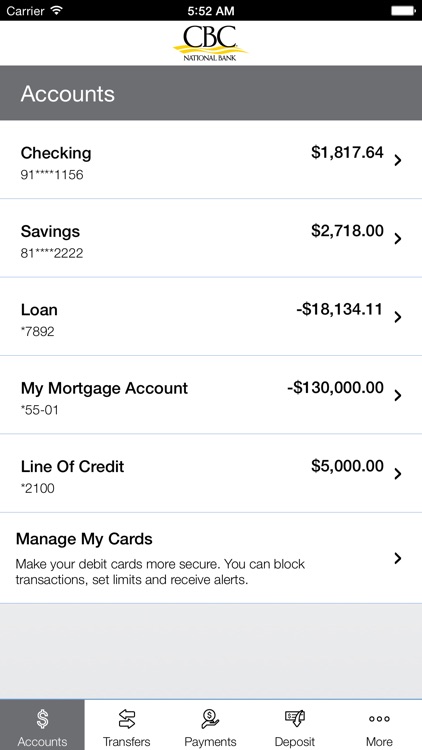The image is a vertical, rectangular screenshot from a cell phone banking app. At the very top, there is a thin horizontal black banner displaying the carrier information on the left corner, a Wi-Fi signal icon, the current time "5:52 AM" in the center, and a battery icon on the right side. Just below this, there is a slightly wider white background banner prominently displaying "CBC National Bank" in the center.

Further down, a gray horizontal banner features the word "Accounts" in white text. Below this, on a white background, a vertical listing of various accounts and their balances is displayed. The accounts include:

1. **Checking**: $1,817.64
2. **Savings**: $2,718.00
3. **Loan**: -$18,134.11
4. **My Mortgage Account**: -$130,000.00
5. **Line of Credit**: $5,000.00

Additionally, there is a section titled "Manage My Cards" with a description encouraging users to enhance the security of their debit cards by blocking transactions, setting limits, and receiving alerts. 

At the bottom of the screen, a navigational row offers more options, including **Accounts**, **Transfers**, **Payments**, **Deposits**, and an additional **More** section.